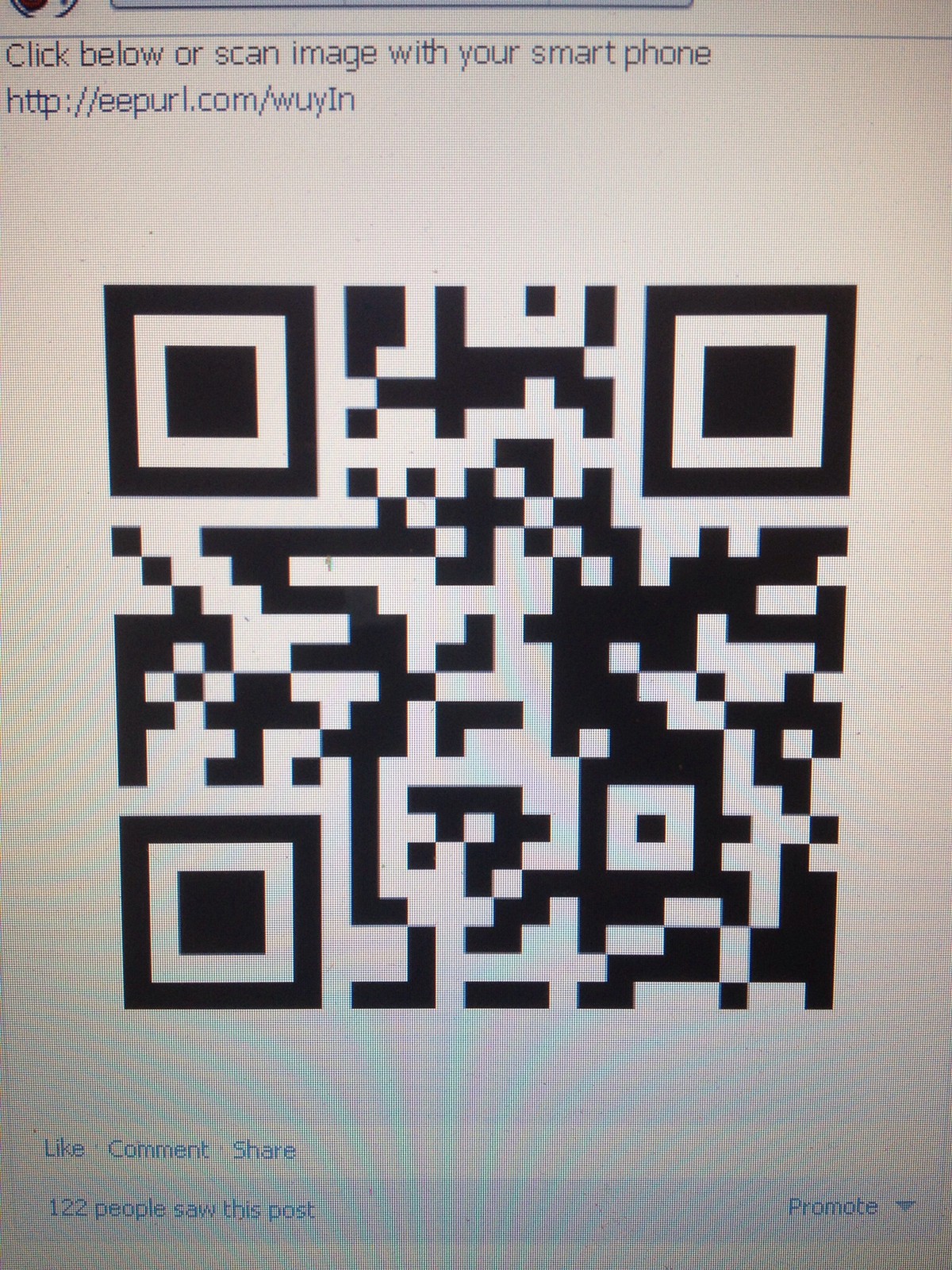The image is a screenshot prominently featuring a very large black-and-white QR code in the center. At the top of the image, in black text, it says, "Click below or scan image with your smartphone," with the website address "http://eepurl.com/WUYIN" displayed underneath. Above this text, a blue line stretches from left to right, with a circular icon partially visible on the upper left corner and the bottom edge of a rectangle slightly showing at the top, adding to the pixelated and somewhat out-of-focus nature of the screenshot. At the bottom of the screenshot, there's a white bar containing options to "like," "comment," and "share" the post. Below this white bar, another light blue line indicates, "122 people saw this post." In the far right corner, a clickable arrow with the text "promote" suggests a drop-down menu option. The overall image appears to be a close-up, slightly distorted capture, likely taken from a smartphone.